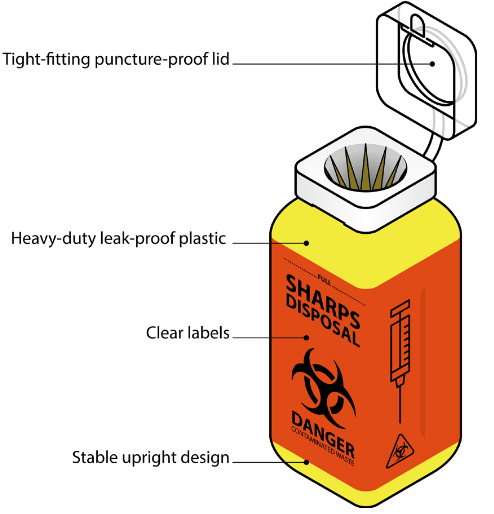This illustration depicts a detailed diagram of a sharps disposal container commonly found in laboratories and doctor's offices. The container is yellow with a red label encircling it, and features black text and symbols for clarity. At the top, a white cap labeled "Tight Fitting Puncture-Proof Lid" is shown partially open, revealing an additional yellow design inside. The main body of the container, labeled "Heavy Duty Leak-Proof Plastic," is yellow and sturdy. 

A prominent red band across the middle of the container carries the words "SHARPS DISPOSAL" in bold, black letters, accompanied by a danger symbol – a biohazard sign – and the word "DANGER" underneath it. On the side of the container's label, a black drawing of a syringe points downward, highlighting its intended use. Below the syringe, nested within a triangle, is another biohazard symbol.

Annotations indicate various features of the container: "Clear Labels" pointing to the text on the red band, "Stable Upright Design" pointing to the container's base, ensuring it's less likely to tip over. The illustration, done in color with black outlines, emphasizes the container's practical attributes, making it a valuable tool for educational materials, brochures, or websites aimed at healthcare providers.